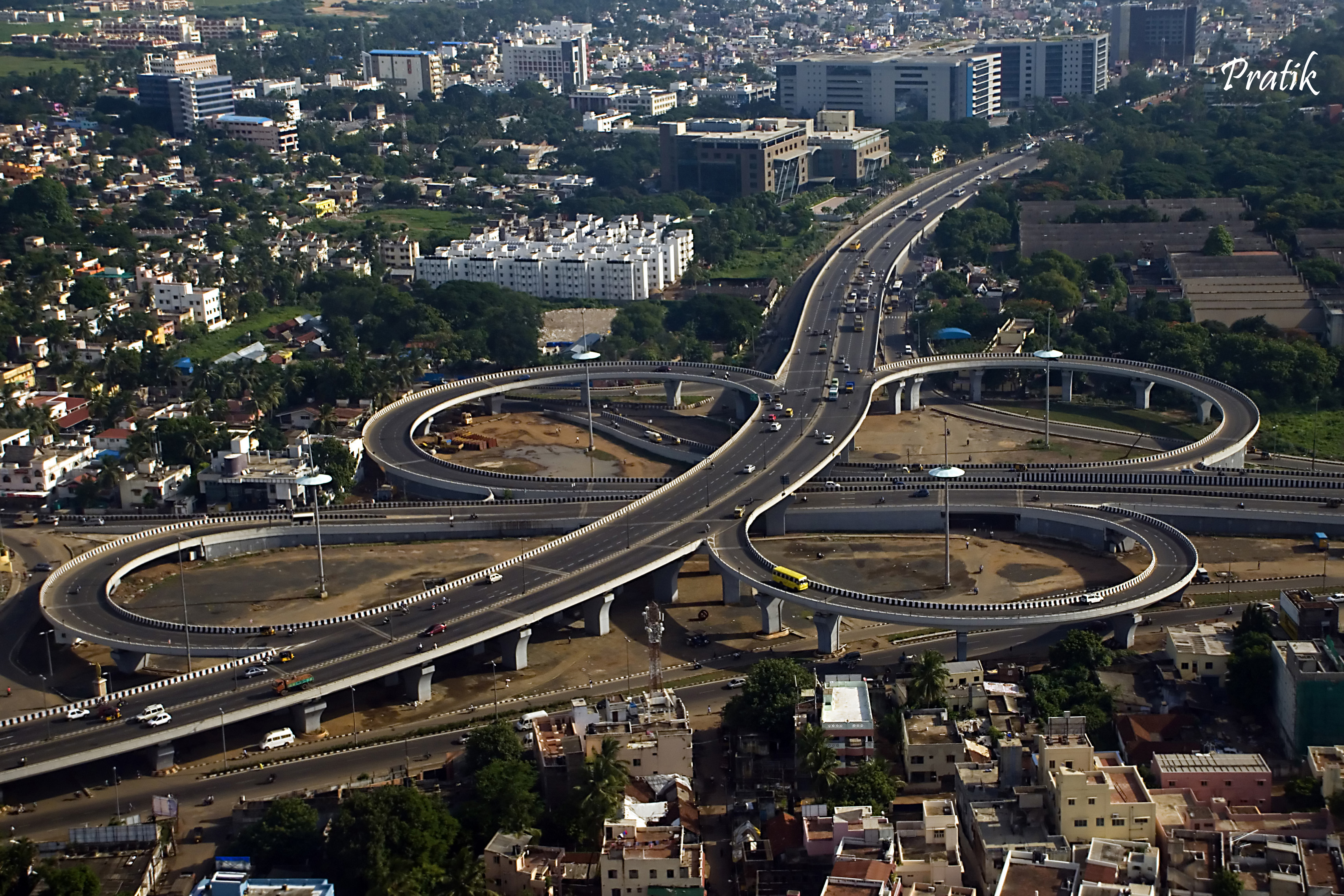An aerial photograph captures a sprawling highway system, likely from Los Angeles, taken from a high vantage point, possibly a helicopter, a few decades ago. The focus is on intricate, cloverleaf interchanges—gray with white accents—that wind elegantly near a cluster of residential buildings. These overpasses create a striking four-leaf clover pattern, framing the scene. The highway, dotted with vintage vehicles including a school bus, a dump truck, and various older model cars, snakes its way through an urban setting. The image transitions from residential zones lined with lush green trees to a burgeoning commercial area in the upper right corner, where larger, more modern buildings rise against the horizon.